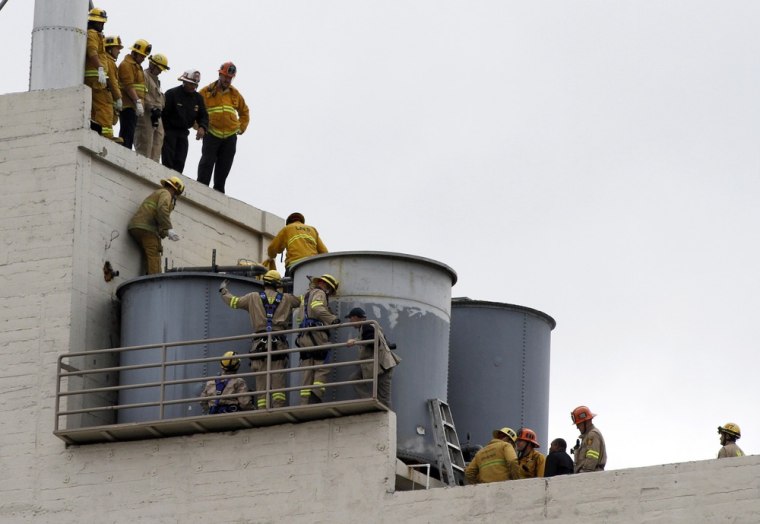The photo captures a light overcast sky serving as the backdrop for a terrace-like building painted in white or beige brick. Positioned at the top of the structure are six men; five wear yellow hard hats and matching yellow hazard or safety suits, while one man dons a police hat and a dark blue or black suit. On a lower level, two individuals, also in yellow hard hats and hazard suits, stand on large, gray cylindrical structures, possibly containers for hazardous material. Another group of three men, similarly attired, is positioned further below. Additionally, there's a leaning ladder against one of the cylindrical structures, where another four or five men in yellow hard hats and safety suits are visible. The scene suggests a coordinated effort among what appear to be construction workers or potentially firemen at a gas plant or factory. The men engage in various activities, some looking downward, others conversing, against the building's tiered levels and the dull, gray sky.